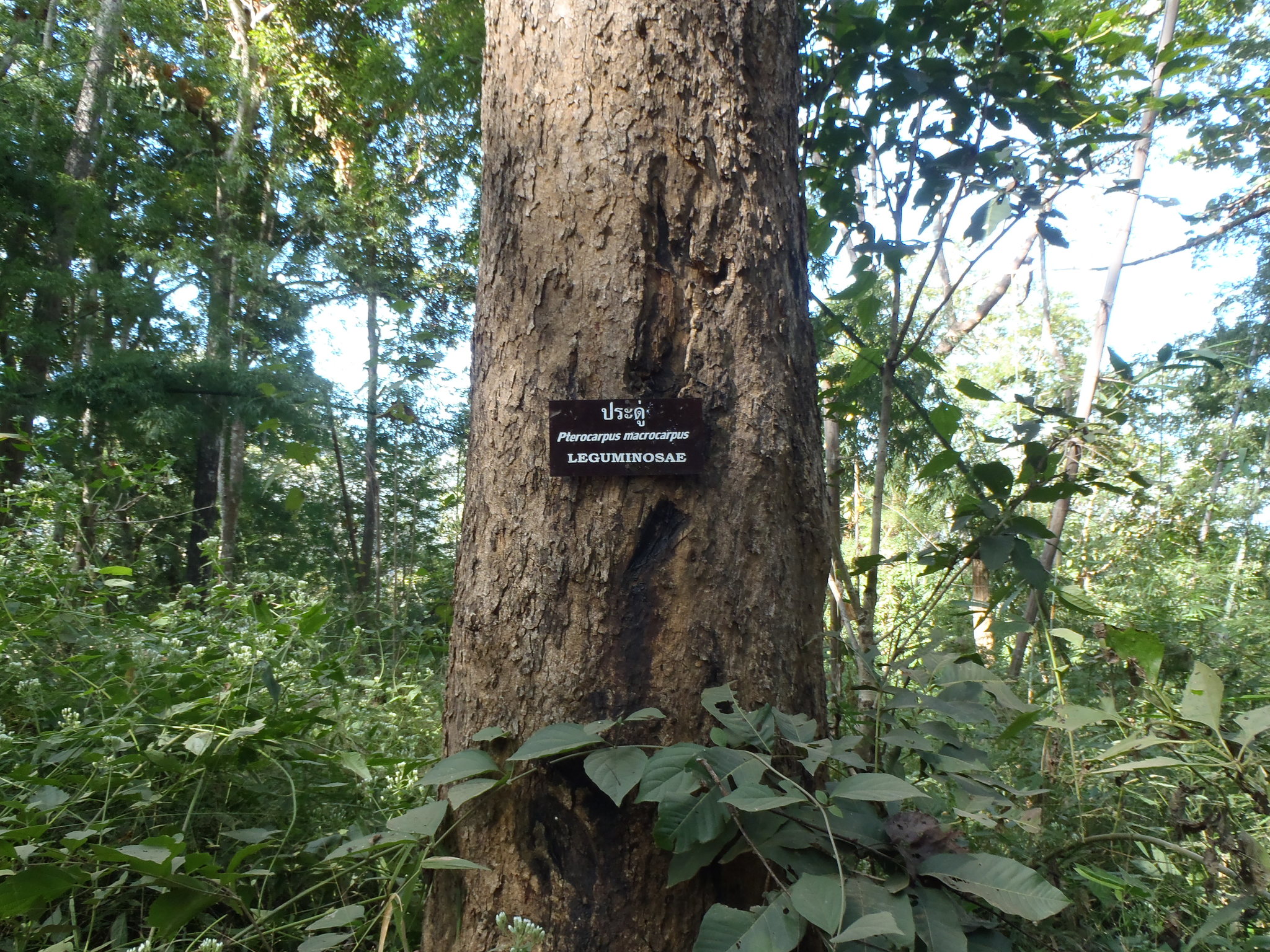The image captures a captivating forest scene, depicting a large, prominent tree at its center. The tree, likely a notable specimen in a conservation park, is identified by a brown signboard affixed to its trunk. This sign features an upper section with unreadable symbols or foreign text, possibly Thai, and below that, Latin text stating "Phosphoropis marcopis." This is followed by the term "Leguminosae," indicating the tree’s classification. The tree is thick and sturdy, surrounded by small, possibly dying plants and vines. In the background, thinner trees with visible foliage extend towards a bright sky, although the sky’s color is ambiguous, appearing either white or possibly cloudy. The scene is lush and verdant, with sunlight filtering through the leaves, creating a vibrant yet serene atmosphere.